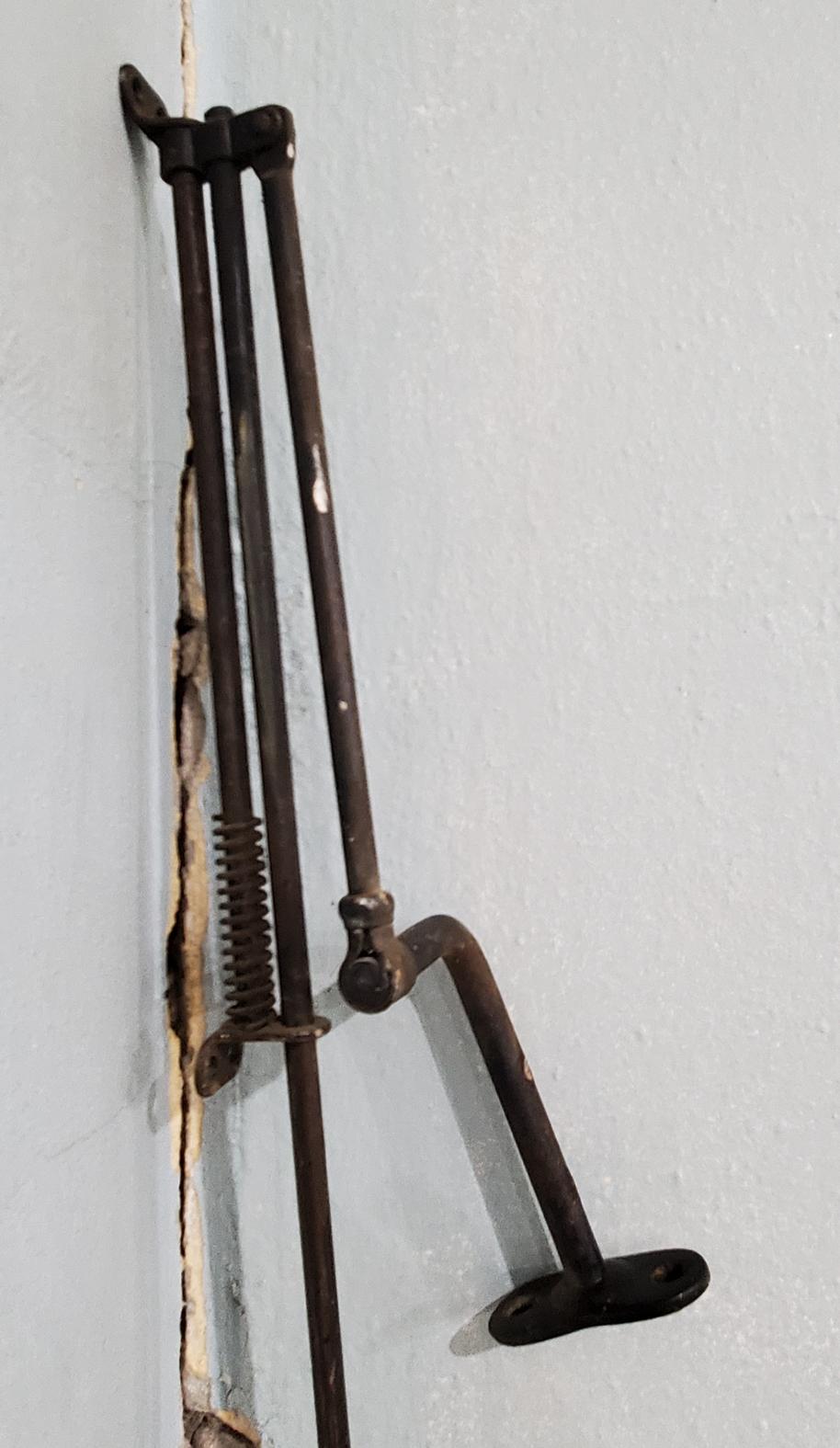The image depicts an old, rusty mechanical tool, possibly used for construction or demolition, leaned against a dilapidated white-bluish wall with noticeable cracks and damage in the corner. The device consists of three thin, long cylindrical rods or poles, with the middle rod being the tallest. The leftmost rod features a spring mechanism at its bottom, while the rightmost rod has a lever or crank handle shaped like an L, which appears to be adjustable. The design suggests that if the rods were straightened, they would form a single, longer piece. Just below the rods, a wrench head can be seen protruding from a hole at the bottom of the image, connected to the construction theme. The tool appears to have a swivel piece at the top, adding to its mechanical complexity. The overall impression is of an old, possibly mid-20th-century device that has seen extensive use.